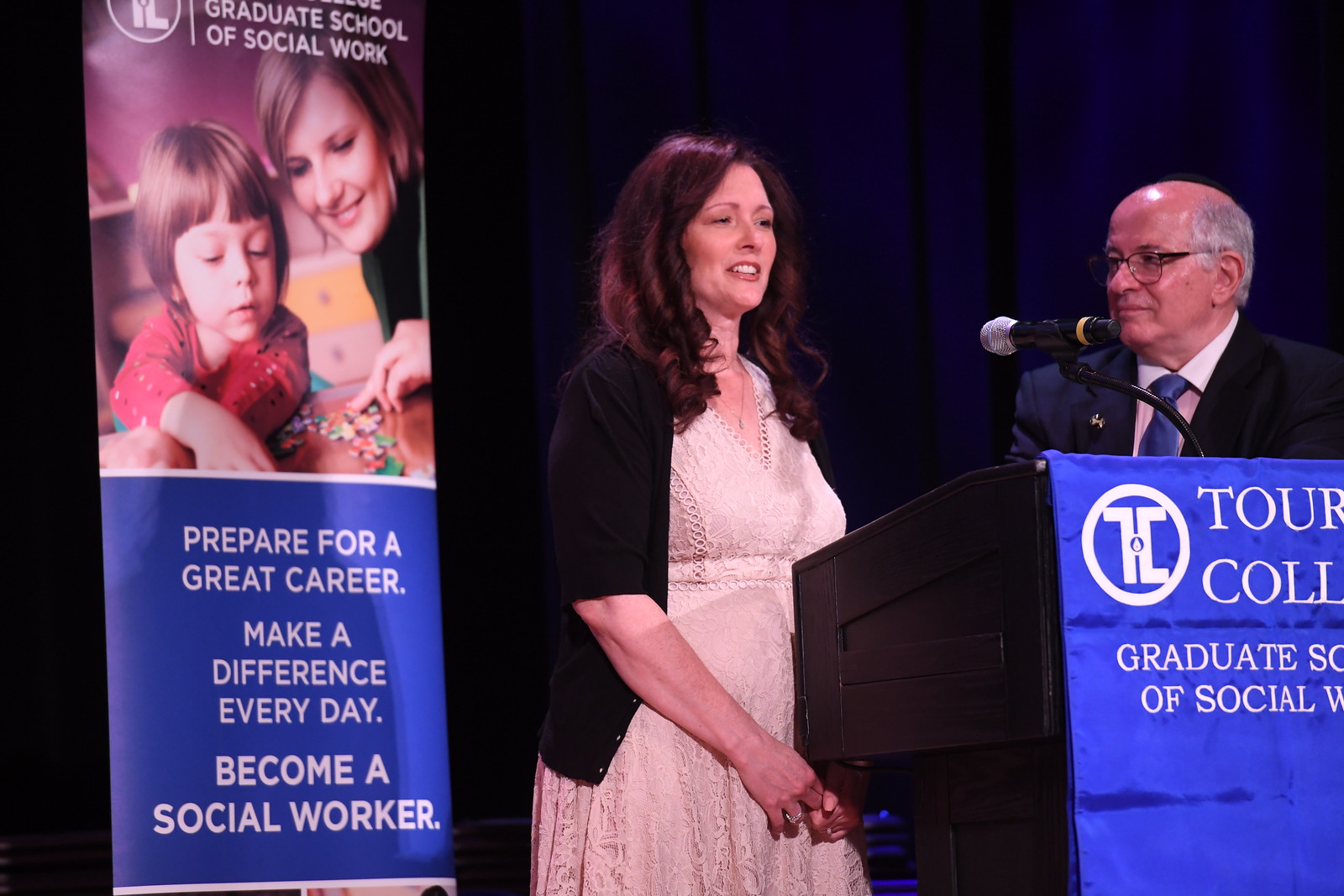In the photograph, two individuals stand at a dark brown podium, adorned with a blue banner reading "Graduate School of Social Work." The banner also partially displays the text "Tour Coll", indicating the name of the college. The woman behind the podium, speaking into a microphone, wears a black sweater over a white dress and her shoulder-length brunette hair is softly curled. To her right, an older man, likely in his 70s, stands with gray hair, glasses, and a blue suit coat paired with a blue tie. Behind them, a larger banner reads: "Prepare for a great career, make a difference every day, become a social worker." The background is a deep, possibly black or very dark blue, giving the scene a formal tone. The man appears to be presenting or supporting the woman, who might be receiving an award or diploma, as they engage with an unseen audience.